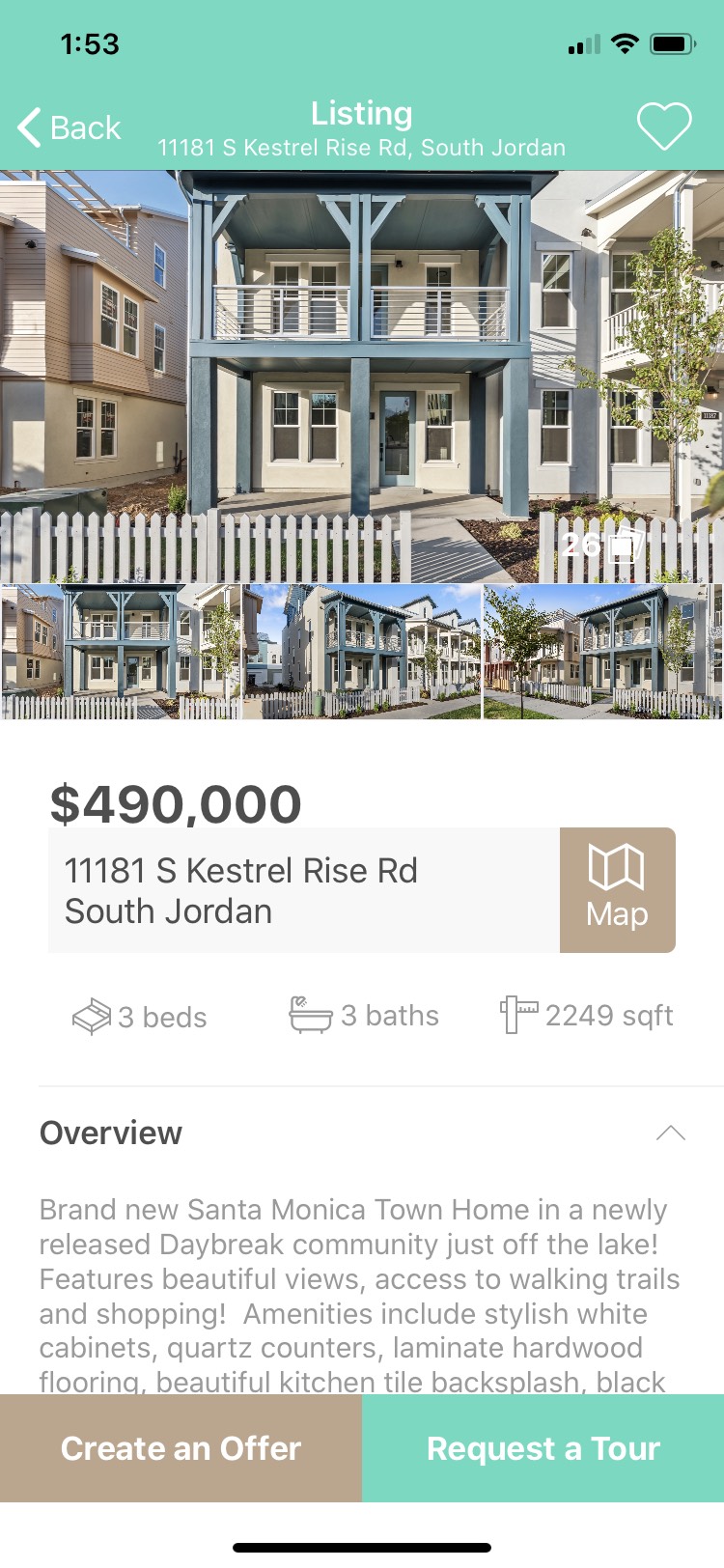The screenshot showcases a real estate listing website with a distinct mint green background. At the top left corner, the time displayed is 1:53 in black text, accompanied by standard mobile icons for signal strength, Wi-Fi, and battery percentage. 

Directly below, the header reads "Listing" in white letters, flanked on the left by a left-pointing arrow labeled "Back" and on the right by a white-outlined heart icon. In the center, the address of the property, "11181 South Kestrel Rise Road, South Jordan," is prominently displayed.

The main image features a two-story house with a cream-colored exterior and blue columns. The house includes balconies on the upper level and an accessible ground floor entrance with no protruding porch.

Below the image, the price of the house is listed as $490,000. Additional information notes the property has three bedrooms, three bathrooms, and spans 2,249 square feet. Two interactive buttons at the bottom offer potential buyers the options to "Create an Offer" or "Request a Tour."